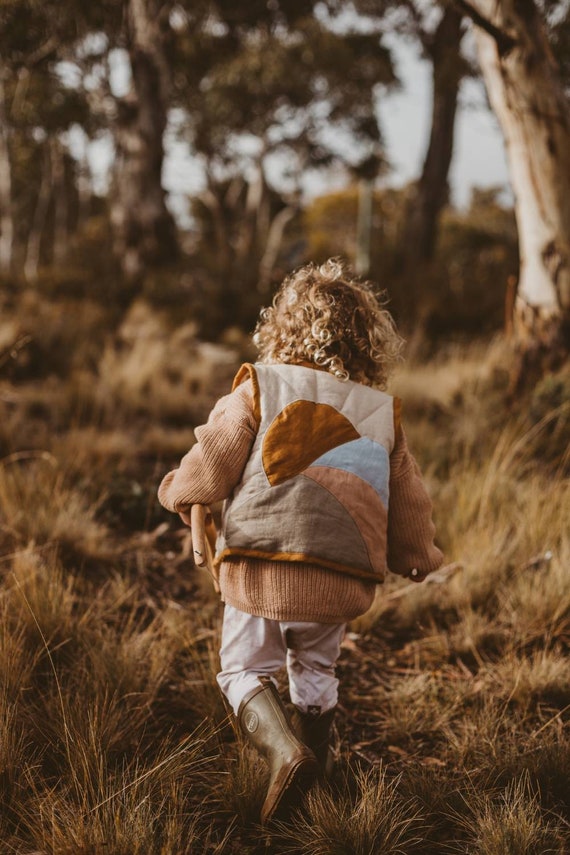The image captures a serene outdoor scene likely during the daytime, possibly at sunrise or sunset due to the lighting. Dominated by a tall, dry area adorned with yellowish and golden grasses interspersed with darker brown accents, it presents a natural, earthy palette. The background showcases blurred, gray-trunked trees, with one prominently whitish from the sun’s rays, coming from the left. A vast bluish sky crowns the background, enhancing the tranquility.

At the heart of the picture, a young girl with long, blonde, curly hair walks forward, her back facing the camera. She appears to be navigating through the tall grass, possibly at a quick pace, suggesting she might be playing or moving away from the photographer. Her attire suggests a cold season – either approaching winter or fall – dressed warmly in a puffy vest bearing a distinctive gold circle with a blue and red curve to the right. Beneath the vest, she wears a vibrant orange knit sweater paired with white pants and black rubber boots, contrasting with the dry, brown surroundings. The overall scene is a warm, visually rich depiction of a young child exploring a peaceful, autumnal landscape.